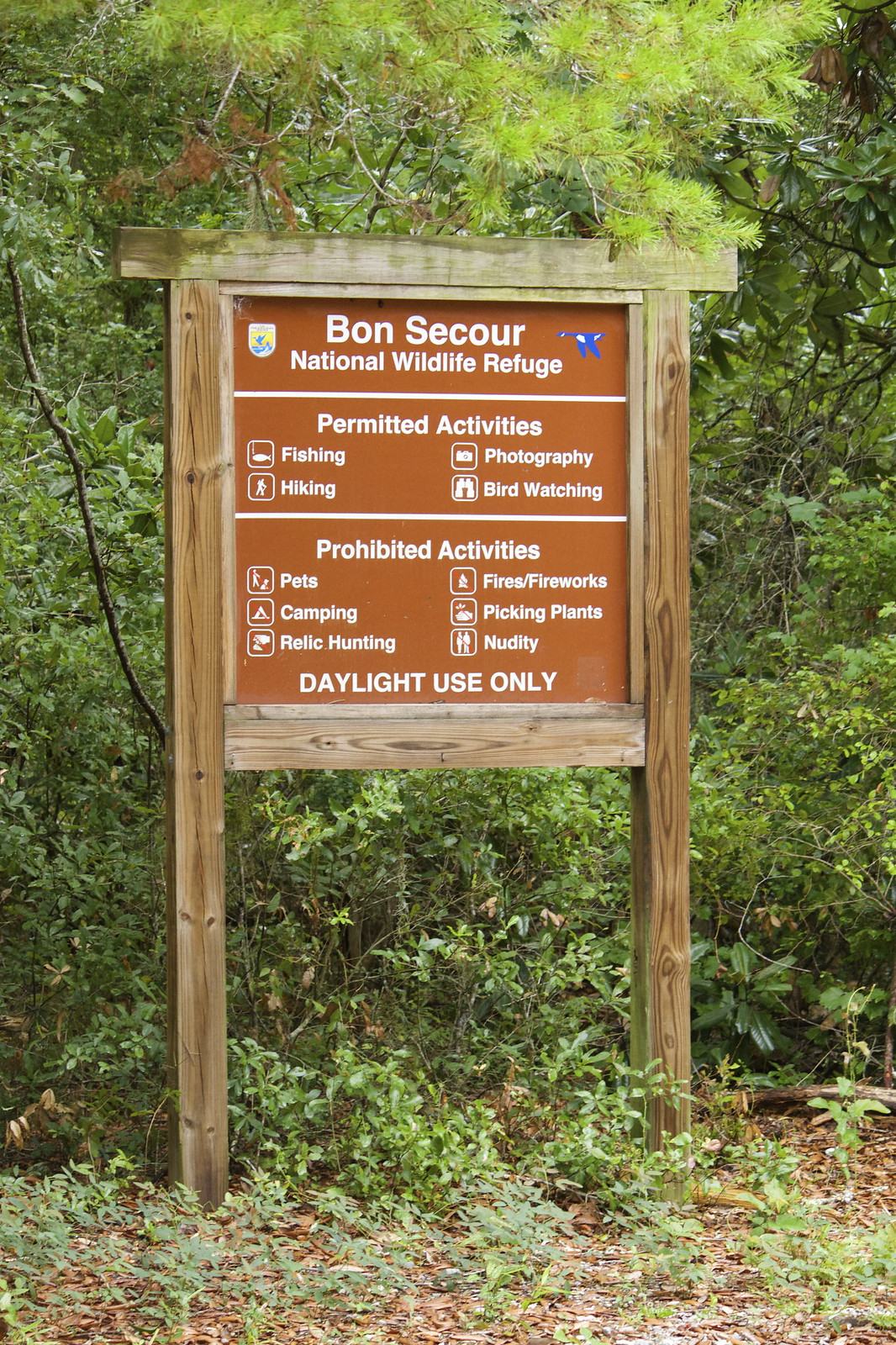This photograph, set in a sunlit, wooded area, captures a detailed wooden-framed sign marking the entrance to Bon Secours National Wildlife Refuge. The sign, mounted between two sturdy four-by-four wooden posts, features a brown background with white text. At the top, the sign reads "Bon Secours National Wildlife Refuge," flanked by graphics on either side. Below this title, a white line separates it from a list of permitted activities: fishing, hiking, photography, and bird watching, each paired with corresponding icons—a fish, a walking person, a camera, and binoculars. Another white line divides this section from the prohibited activities: pets, camping, relic hunting, nudity, picking plants, fires, and fireworks, each indicated by appropriate graphics, such as an animal for pets and a tent for camping. At the very bottom, it specifies "daylight use only." The background teems with lush green bushes, while the foreground features brown soil and lower vegetation, enhancing the natural, serene setting of the refuge.